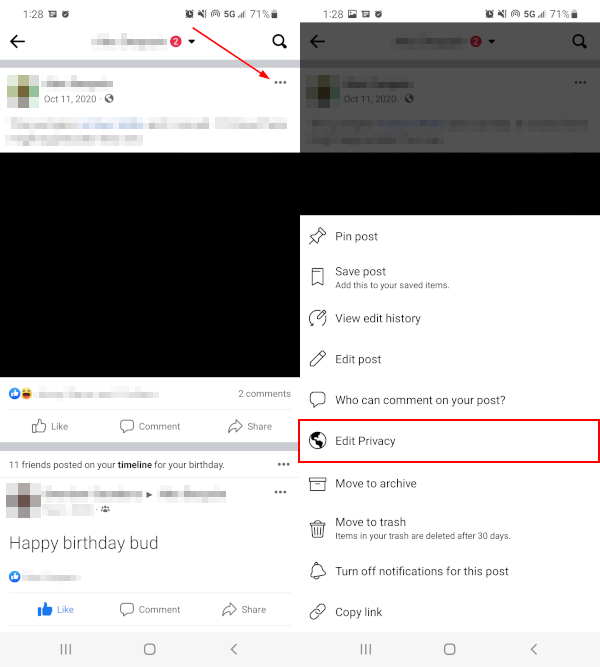A detailed caption for the screenshot could be:

"This image is a screenshot of a Facebook page viewed on a smartphone, as indicated by the visible icons for battery life, 5G data, and various notifications at the top. The screenshot was taken on October 11, 2020, as noted in one of the posts. The main part of the screen is divided into a two-panel display with two pictures side by side, although the right picture is partially obscured by an active pop-up menu. The pop-up menu offers several options: Pin Post, Save Post, Add This to Your Saved Items, View Edit History, Edit Post, Who Can Comment On Your Post, Edit Privacy (highlighted with a red outline), Move to Archive, Move to Trash, Turn Off Notifications for This Post, and Copy Link. Below this, there is a post with a like button, a happy face reaction, and two comments. Another part of the screen shows a message stating, '11 friends posted on your timeline for your birthday,' with one visible post saying, 'Happy Birthday, bud,' accompanied by one like. Other elements on the screen, such as additional text, are grayed out and unreadable."